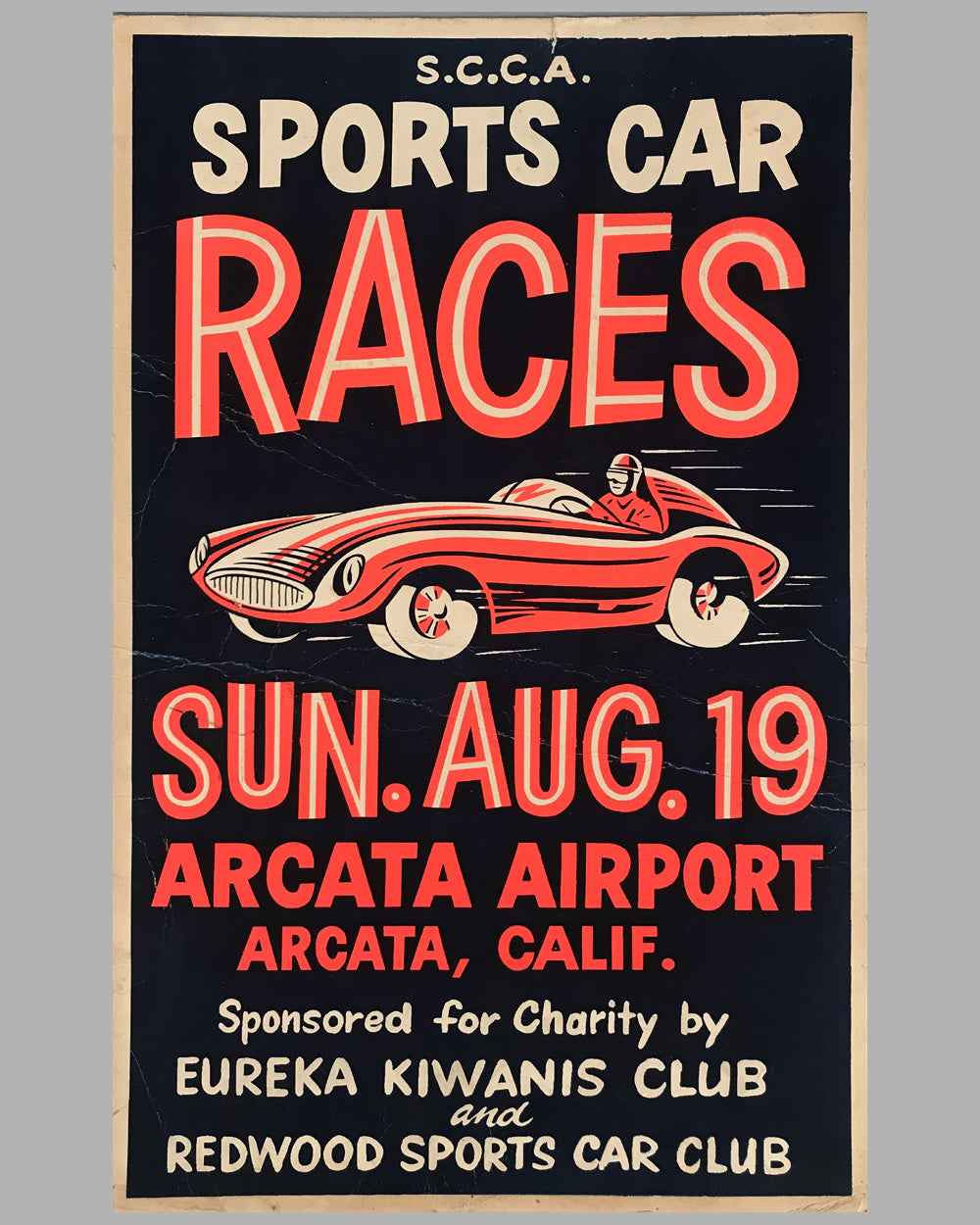This image depicts an advertisement for SCCA (Sports Car Club of America) sports car races. The poster features a vintage design with a black background, highlighting text in white and a subtle reddish color. Dominating the center of the poster is a drawing of an old-timey sports car, with a long hood, a small windshield, and a protective dome behind the driver, mimicking classic race car aesthetics. The text announces the event date, "Sunday, August 19th," although the year is not specified, and the location is Arcata Airport in Arcata, California. The event is sponsored for charity by the Eureka Kiwanis Club and the Redwood Sports Car Club. This booklet-style poster measures approximately 2 by 5 or 3 by 5 inches and does not include any images of people.